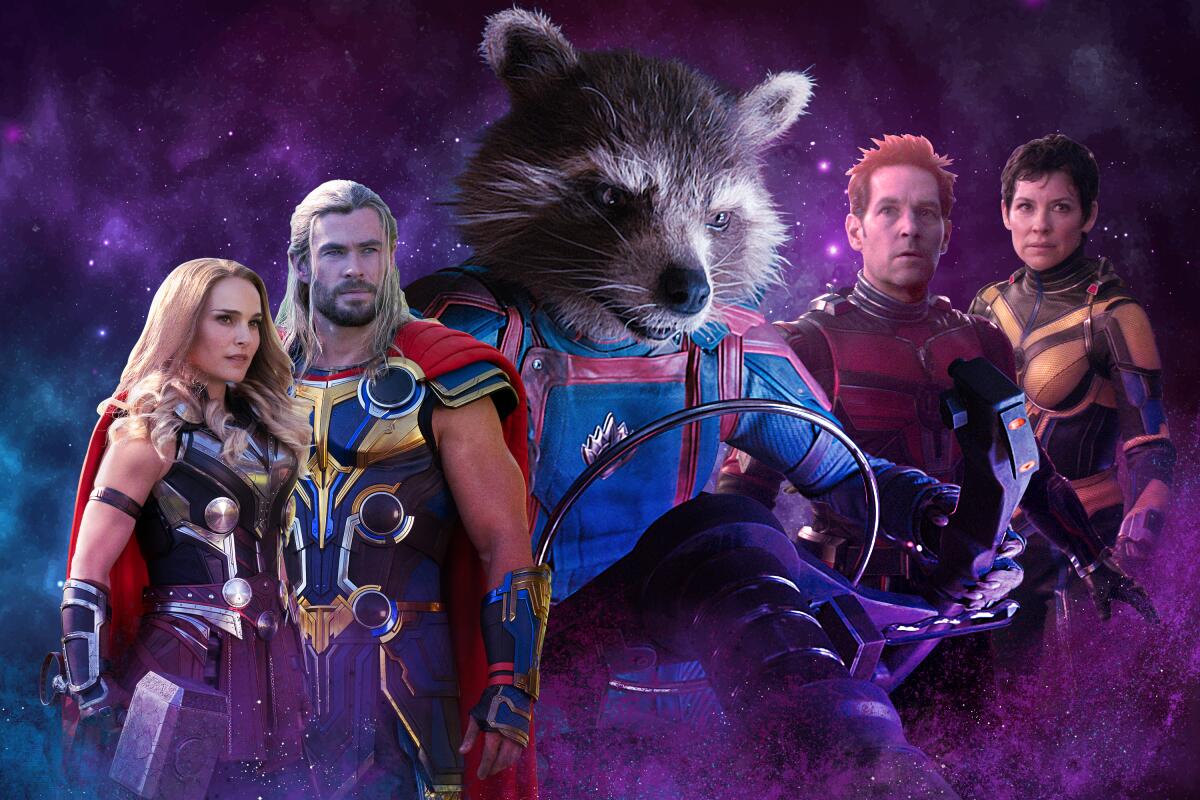This vibrant collage features an array of famous Marvel superheroes set against a cosmic backdrop with hues of purple and blue, sprinkled with twinkling stars. Central to the image is Rocket Raccoon from Guardians of the Galaxy, distinguished by his large head, black and white fur, and mischievous smile. Rocket is donned in his signature leathery blue outfit accentuated with red lines, gripping a silver steering wheel, suggesting he's poised on a spacecraft or motorbike. Flanking him are other iconic characters: to his left stands Thor (likely Chris Hemsworth) in his classic yellow and blue armor with a red cape, alongside a woman in dark armor, possibly Valkyrie, identifiable by her medium-length blonde hair and the formidable hammer in her grasp. To Rocket's right, Paul Rudd appears in an unspecified red superhero outfit, accompanied by another female hero clad in a striking gold and orange suit sporting short black hair. This ensemble of heroes, none of whom share a common movie universe, evokes a powerful sense of unity amidst the star-studded galaxy backdrop.